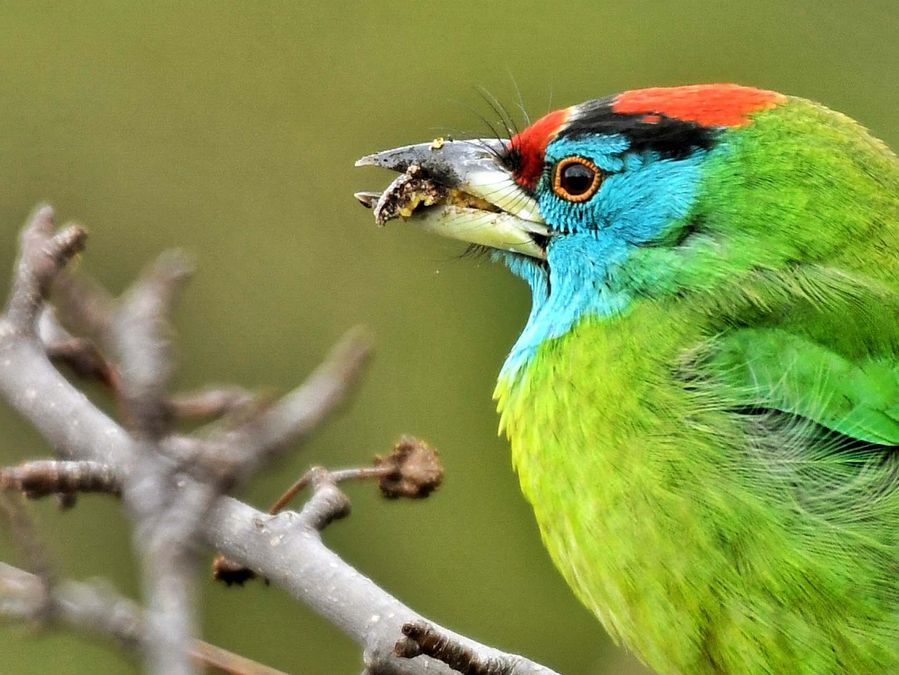This color photograph captures a vibrantly colorful bird known as the blue-throated barbet, native to the foothills of the Himalayas and Southeast Asia. The close-up shot prominently features the bird’s head and neck, perched on a barren branch, while the rest of its body is partially out of frame. Its feathers are a kaleidoscope of colors: a striking red crown, bordered by a black stripe above the eye, transitions into brilliant blue around the eye and neck. The eye itself is black, encircled by a golden ring. The beak, short and sharp, is a mix of black and yellow hues. The visible portions of the bird's body are a luminescent green. In its open beak, the bird holds a grub, its beak smeared with the insect's remains. The background is a blurred mix of brown and green tones, highlighting the bird's vivid plumage even more. The overall scene suggests a moment in the wild, captured with exceptional clarity and detail.